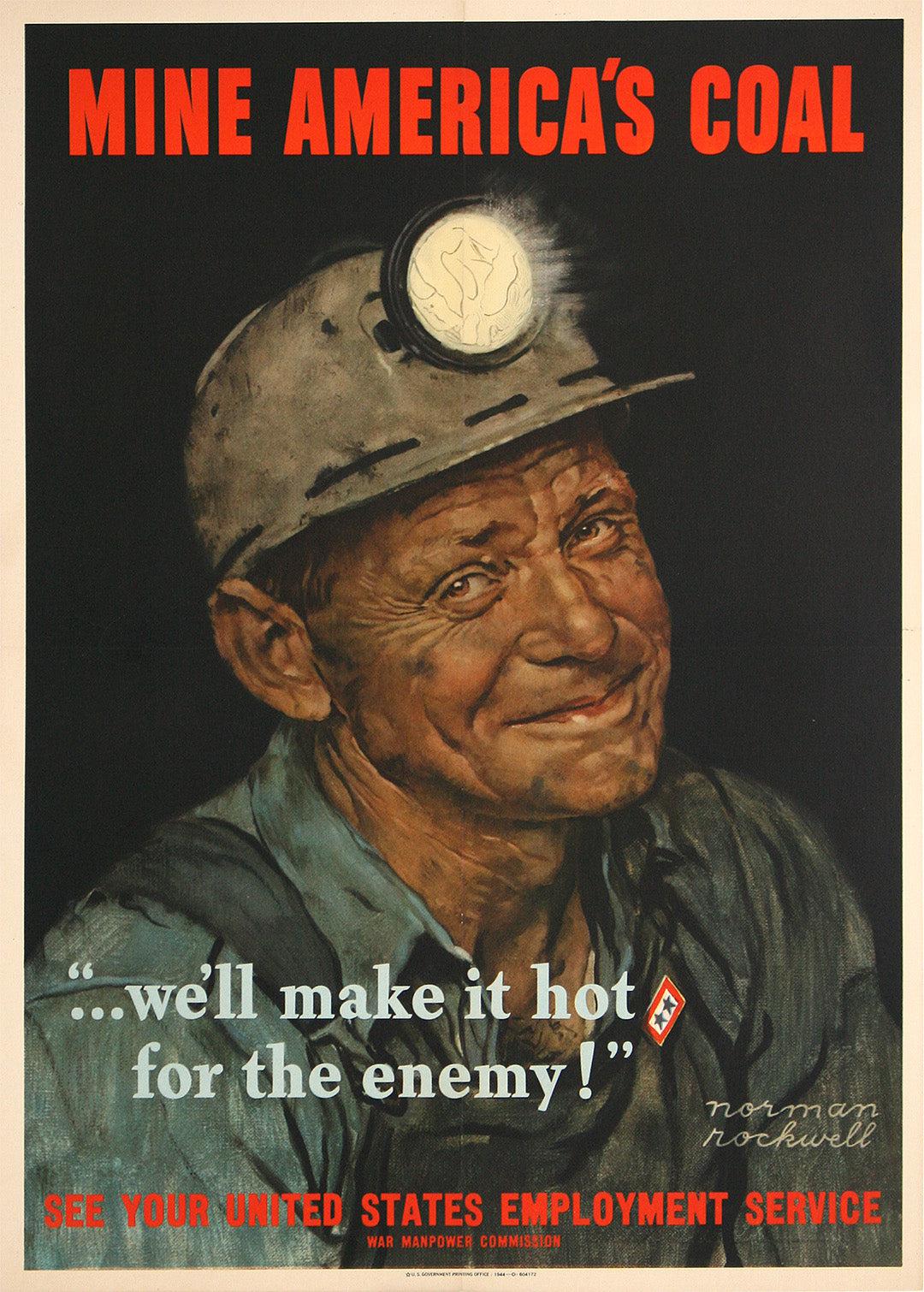This full-color artistic image, rendered by Norman Rockwell, features a vertically rectangular composition with an off-white border encasing a predominantly black background. The focal point is an older Caucasian man with a wrinkled, worn face, signifying a life of hard labor. He dons overalls and a miner's helmet equipped with a lamp, his demeanor one of steadfast resolve as he gazes slightly to the left with a subtle, closed-mouth smile. The text prominently displayed across the top in bold red all-caps reads, "MINE AMERICA'S COAL." Below, within quotation marks in white, it declares, "We'll make it hot for the enemy." At the very bottom, it prompts, "See your United States Employment Service," also in red. Additionally, a note at the bottom mentions the "War Manpower Commission," indicating the image's wartime recruitment purpose. This piece, evocative of a vintage advertisement or magazine cover, promotes coal mining as a patriotic duty during war times.